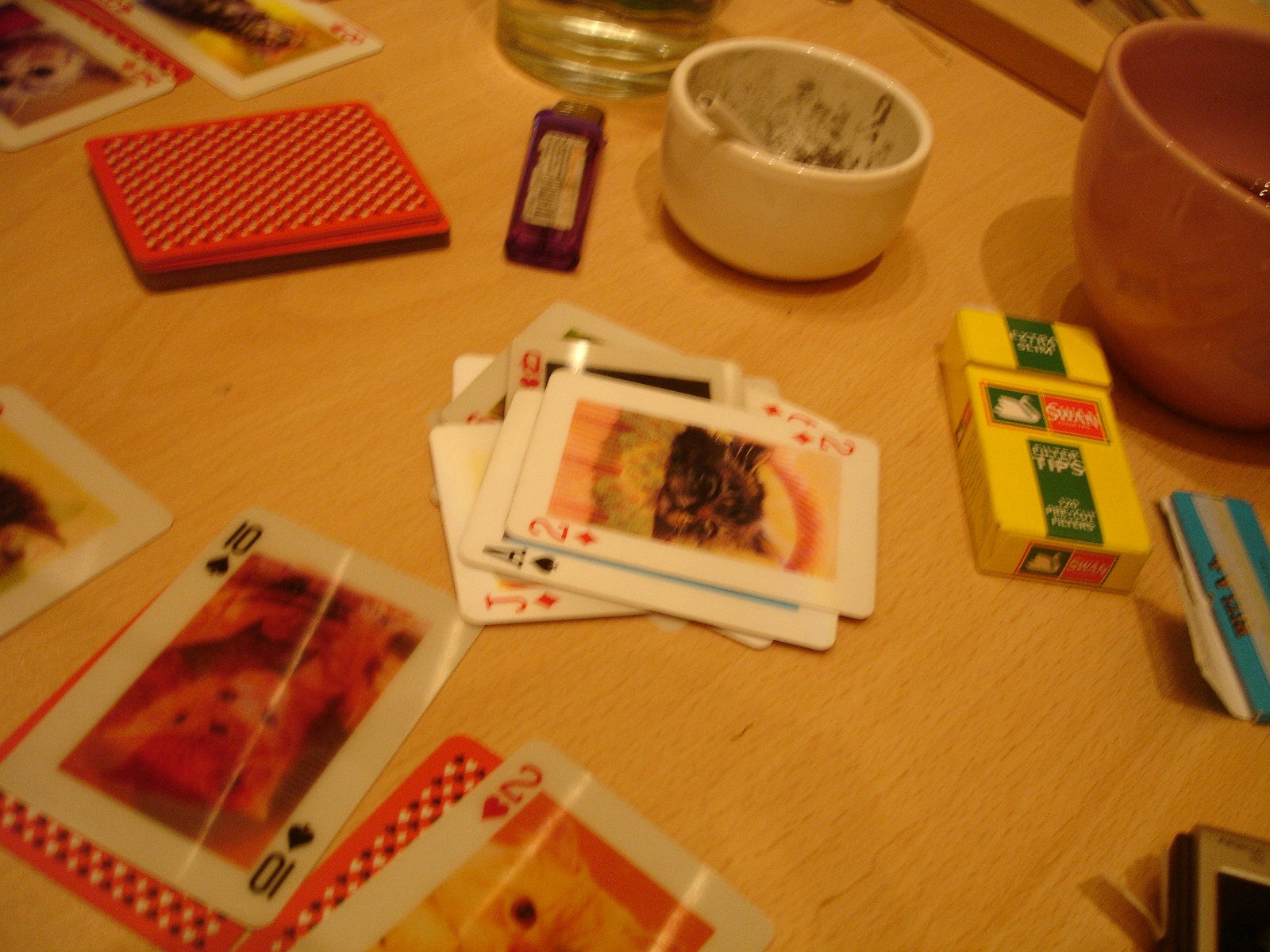This photograph, though slightly blurry, captures a scene of casual leisure on a light brown wooden table that is slightly angled toward the right. A spread of playing cards is situated predominantly in the lower left corner, with some cards face up revealing illustrations of cats, resting atop a pile of face-down cards showcasing red and white patterned backs. In the center of the table lies another stack of face-up cards, while to the left, a separate pile with the same red and white back design is placed diagonally upward to the right.

A rectangular-shaped purple Bic lighter sits askew near this pile. Adjacent to the lighter on its right is a tall, white porcelain bowl, notable for its round shape and the dark smudges inside, with a straw or potentially a cigarette protruding from its left side.

In the center right, a bright yellow packet of Swan cigarettes lies diagonally, flaunting a green stripe and a vivid label with a white swan in a green and red banner. Completing the scene on the far right is a large orange coffee mug, rounding off this eclectic collection of items that hint at a laid-back, informal gathering.